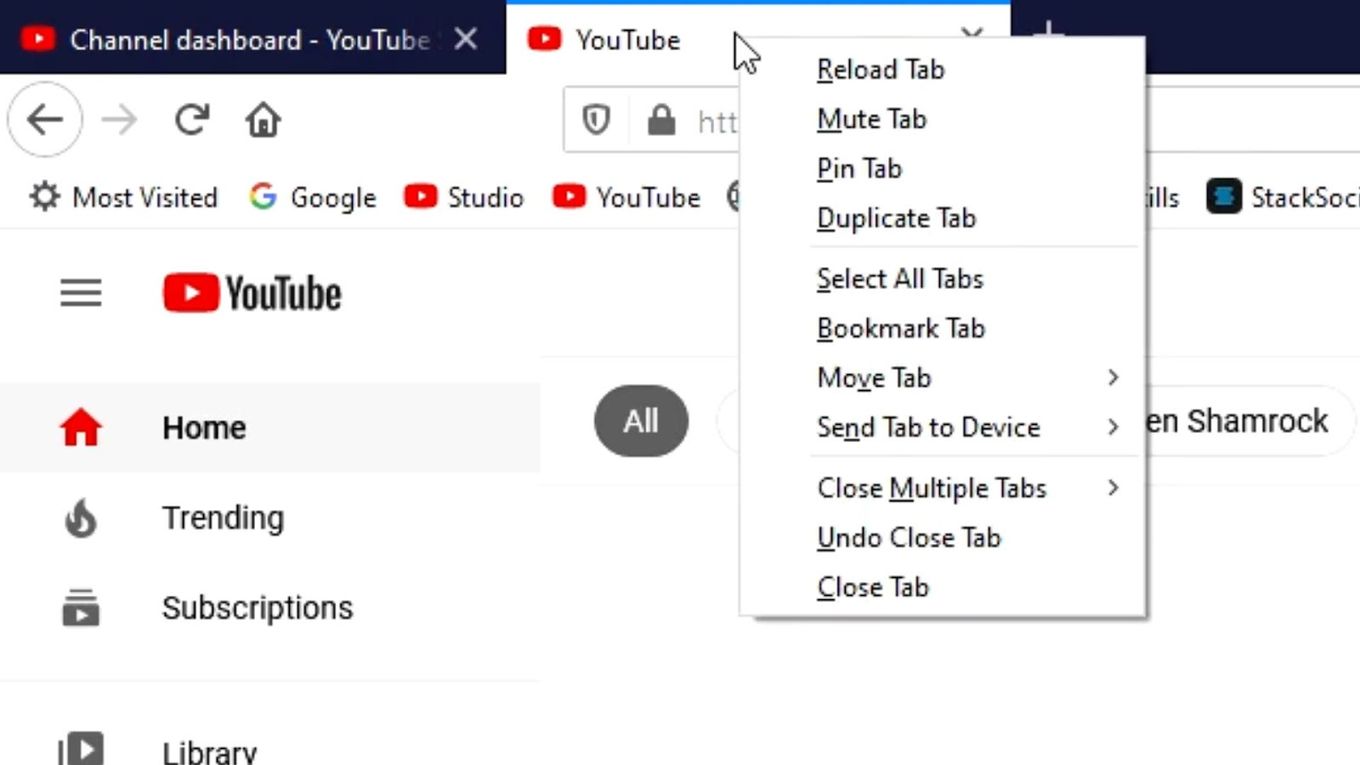The image depicts a detailed view of a YouTube page opened in a web browser. There are two tabs visible at the top of the browser: the first one, labeled "Channel Dashboard from YouTube," and the second one, currently active, is the main YouTube page. The user's mouse is hovering over the YouTube tab, having right-clicked it to reveal a context menu. This menu offers various options including "Reload tab," "Mute tab," "Pin tab," "Duplicate tab," "Select all tabs," "Bookmark tab," "Move tab," "Send tab to device," "Close multiple tabs," "Undo close tab," and "Close tab."

On the homepage, only a partial view is shown. The recognizable YouTube logo is visible, along with several navigation options on the left side: "Home," "Trending," "Subscriptions," and "Library." Additionally, the browser's bookmark bar is partially visible, displaying bookmarks such as "Most Visited," "Google," "YouTube Studio," and "Stack Social," with a few more bookmarks concealed by the options box.